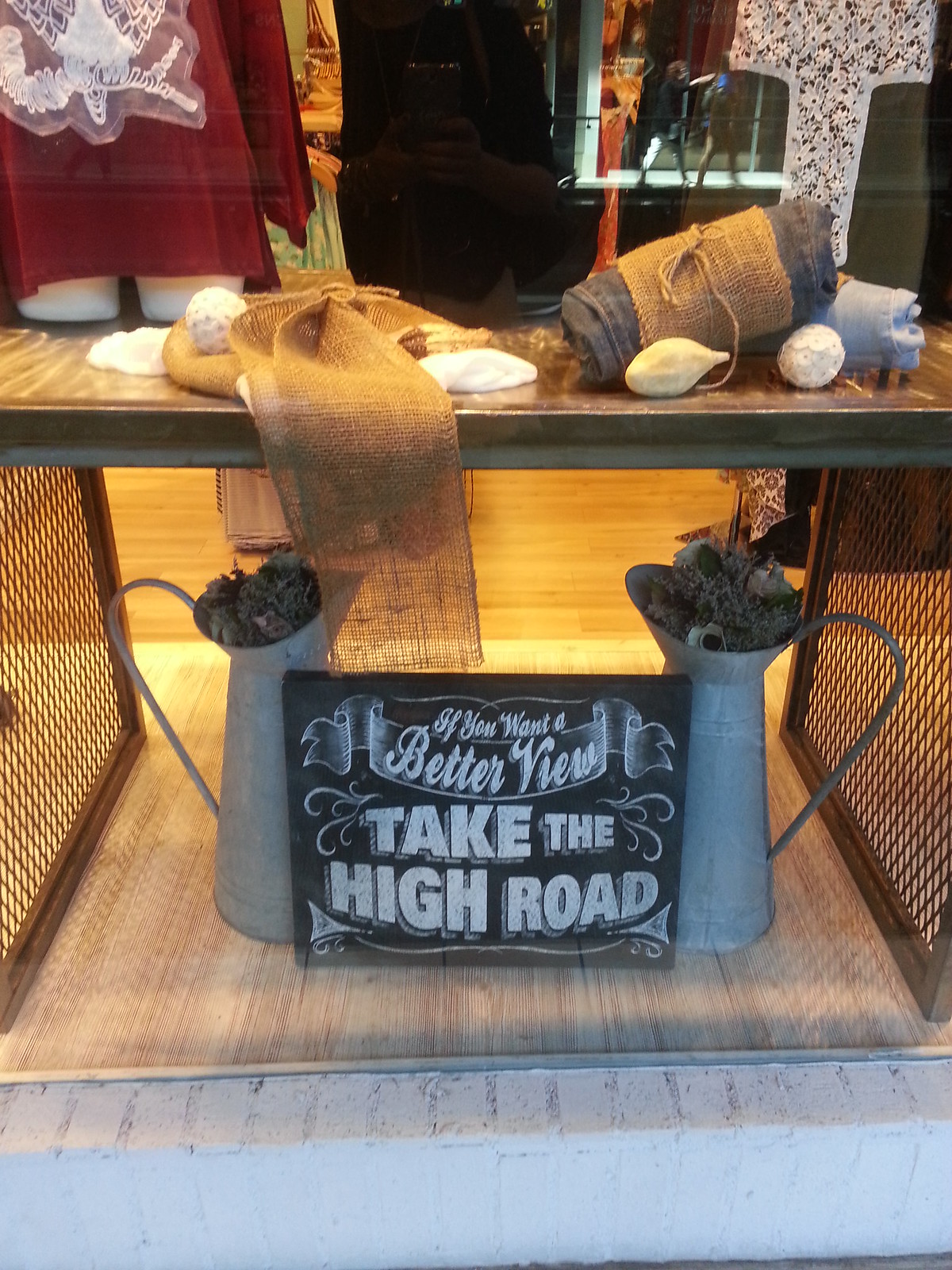The image depicts an indoor scene likely set in a fabric store, thrift shop, or consignment shop. The photograph is framed vertically, with the main focus on a wooden table centered toward the top. The table showcases various decorative items, including a red shirt worn by a mannequin, a colorful scarf, a lamp, and several bulbous fabrics and yarns. Toward the left and right of the table, two large pots filled with pine cones add to the eclectic display.

A distinct visual element is the brick border at the bottom of the image and the reflection of the outside in a large glass pane captured by the camera. Below the table, at the very bottom of the image, a chalkboard-style sign reads "If you want a better view, take the high road," providing an intriguing and whimsical note to the scene. The sign appears beneath some screens and amidst a myriad of other intricate details on the tabletop, surrounded by colors including black, gray, white, brown, tan, dark red, orange, and green.